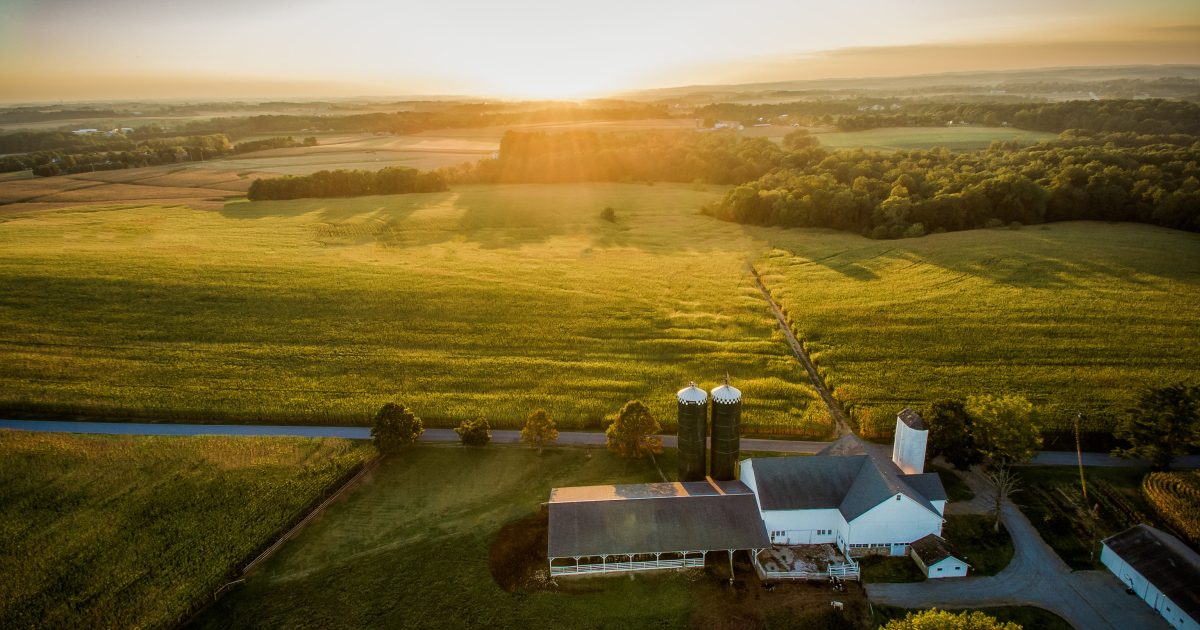This captivating aerial image showcases a serene farming landscape at sunset. The silver and light gray sky subtly transitions to a vibrant central glow, with soft orange clouds decorating the horizon. Rolling hills frame the background, their beauty unmarred by mountains, while lush green trees and scattered farm fields dominate the foreground. 

Centered in the scene is a sizable farmhouse complex, positioned in the lower right-hand corner. The farmhouse itself is distinguished by its white walls and gray roofs. Adjacent to it, there are three silos—two are blue with white caps, and one is white with a black cap. Nearby, there’s a large cattle area characterized by gray roofing and white fencing, suggesting a well-maintained livestock area. An add-on structure, possibly a stable, sits close to the house with open sides and a roof.

A meticulously maintained green yard lies to the left, complemented by expansive green farm fields stretching into the distance. Interconnecting narrow roads weave through these fields, with one prominent road meeting a highway that circles back to the dense grove of green trees in the middle of the expansive farmland. The setting sun casts a warm amber-yellow hue over the entire landscape, creating a picturesque and tranquil farming scene.